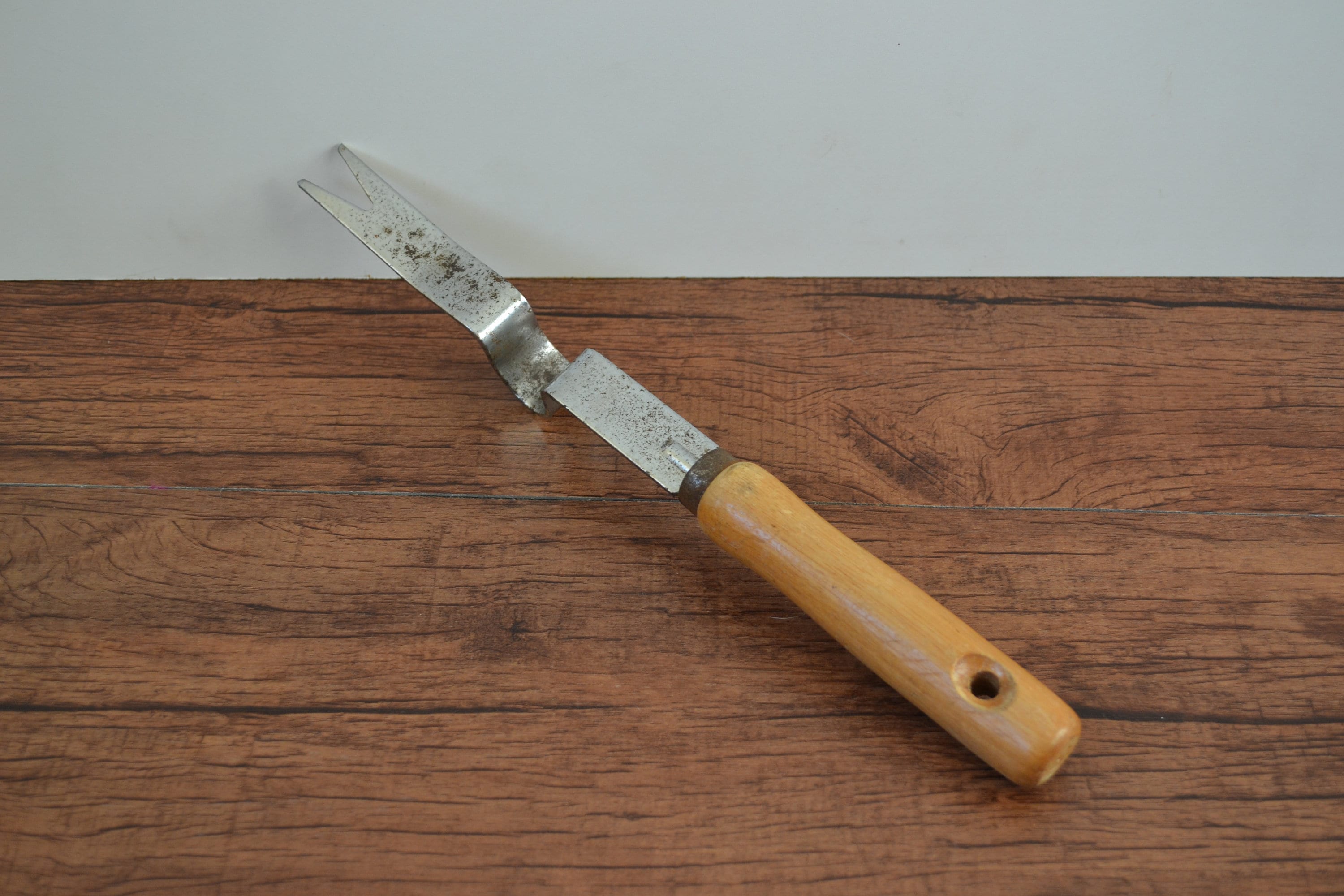The image showcases a construction tool lying across a wooden floor, against a light gray wall where the floor and wall meet. The floor features horizontal wooden panels, stained a darker shade with distinct veiny lines and black streaks. The tool itself has a wooden handle that includes a hole at the bottom, likely for hanging. Attached to the handle is a metal component that extends horizontally, dipping and rising before terminating in a forked end with two prongs. The tool appears to have some dirt on it, possibly indicating it is used for tasks related to painting, flooring, or outdoor work such as dealing with gravel or grass.